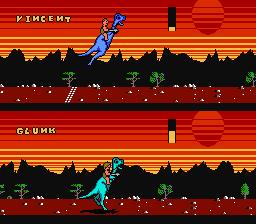The image is a screenshot from a computer game featuring a split-screen display. The upper screen is labeled "Vincent" and the lower screen is labeled "Glunk." The top half shows a young caveman boy riding a blue dinosaur, while the bottom half depicts another caveman boy riding what looks like a baby Triceratops. The vibrant background transitions from orange to red and yellow, evoking the atmosphere of a sunset or a fiery volcanic sky. Silhouettes of mountains or trees are visible in black, interspersed with a few green trees, enhancing the prehistoric landscape. Both screens show rocky terrain with scattered stones or rocks on the red ground. This screenshot captures the simultaneous action experienced by both players in the game.